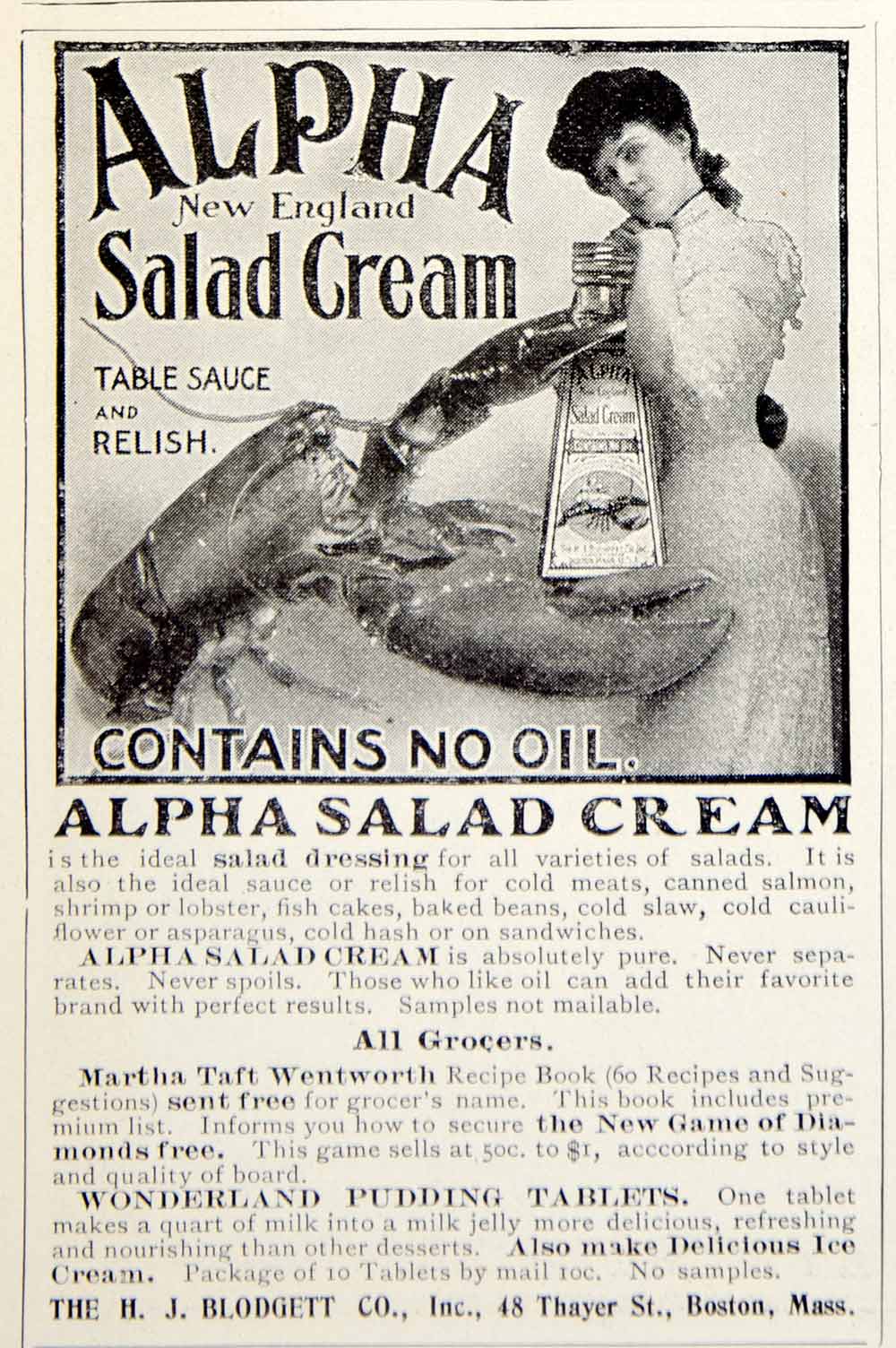This vintage advertisement from around 1900 features a stylish woman in a long white dress, her hair pulled back and adorned possibly with a small bow and a ribbon around her neck, holding a gigantic bottle of Alpha New England Salad Cream. In front of her is a giant crab with its claws gripping the bottle. The ad is framed with a black border. The top of the advertisement displays "ALPHA" in bold black letters, followed by "New England" in gray letters, then "Salad Cream" in black. It also highlights that the product is a "table sauce and relish" and prominently notes "Contains No Oil."

Beneath the main image, the advertisement extols the virtues of Alpha Salad Cream, describing it as the ideal dressing for all varieties of salads, as well as a perfect sauce or relish for cold meats, canned salmon, shrimp, lobster, fish cakes, baked beans, coleslaw, cold cauliflower or asparagus, cold hash, or sandwiches. Additional small print details that Alpha Salad Cream is absolutely pure, never separates, never spills, and never spoils. Those who prefer oil can add their favorite brand for satisfactory results. It mentions "All Grocers" stock the product, along with an offer for the Martha Taft Wentworth Recipe Book containing 60 recipes and suggestions, available for free upon providing a grocer's name. The book also includes a premiums list and information on how to obtain the "new game, diamonds free," priced between $0.50 to $1.00 depending on the style and quality of the board. The ad concludes with details about Wonderland Pudding Tablets—each tablet transforms a quart of milk into a milk jelly or delicious ice cream. The H.J. Blodgett Company, Incorporated, located at 48 Thayer Street, Boston, Massachusetts, is noted as the manufacturer.